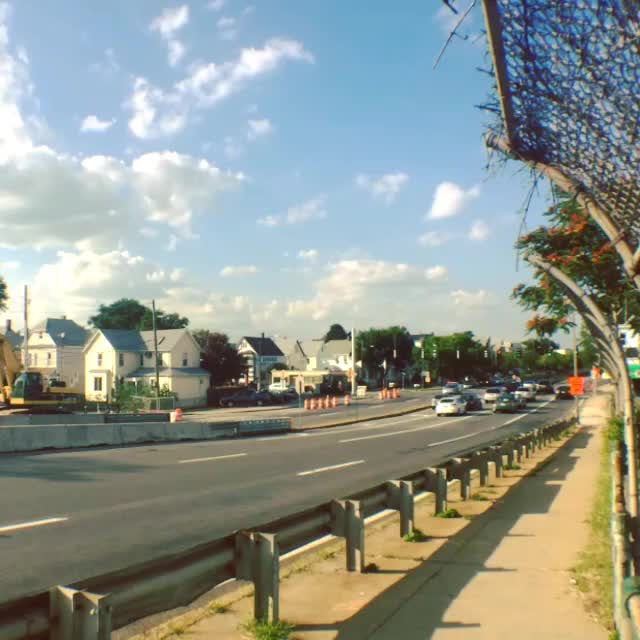This image depicts a divided highway with three lanes in each direction. The majority of the highway is clear of vehicles, but towards the far right of the image, a significant amount of traffic can be seen, potentially halted by a stoplight. To the right of the highway, there is a curved fence, followed by a sidewalk and a guardrail. In the middle of the highway, traffic pylons are visible. On the opposite side of the street, a row of two-story homes can be seen. The sky above is a brilliant blue, adorned with scattered, fluffy clouds.